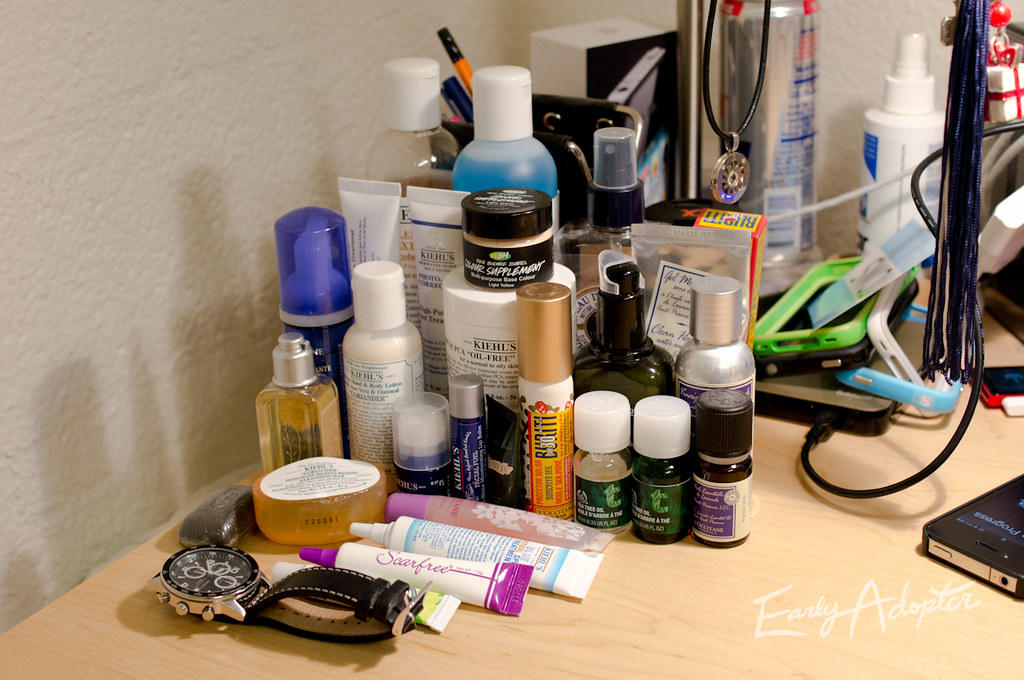A cluttered bedroom dresser top strewn with various personal items under natural lighting. Prominently displayed is a wristwatch placed among several makeup products and skincare oils, suggesting a busy morning routine. A medallion necklace hangs elegantly from the corner, adding a touch of personal style. Scattered around are multiple cell phone bumper cases, indicative of someone who values protecting their device. A graduation tassel dangles nearby, hinting at recent academic achievement. At the back, there's a squirt bottle, likely containing hairspray, positioned next to an energy drink, a Red Bull, signifying a mix of self-care and the need for an energy boost. Behind the necklace and adjacent to the Red Bull, a case for what appears to be an iPhone is visible. At the bottom right, part of an active phone screen is seen, displaying a contact name, suggesting the person is multitasking by speaking on the phone through speaker mode while going about their activities. The image has a caption, "early adopter," adding an element of curiosity and possibly hinting at the owner's penchant for trying out new trends or technology.